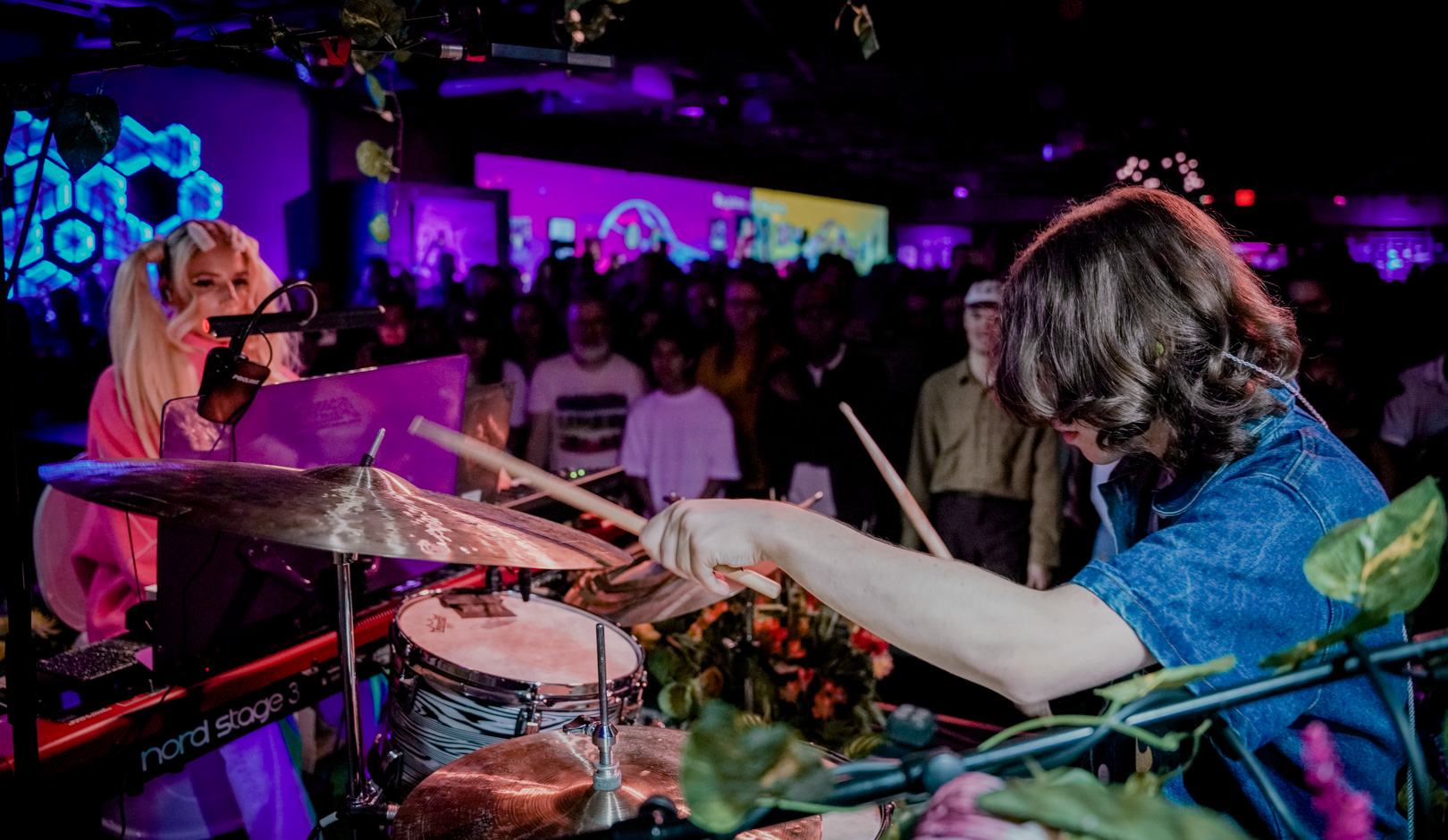In this indoor nightclub photo, a central figure focuses intensely on playing the drums. The drummer has wavy, shoulder-length brown hair nearly obscuring their face and wears a blue denim shirt. Their hands, holding light brown drumsticks, appear in motion as they strike a brass cymbal and a visible drum. To the left of the drummer stands a woman with long blonde hair styled in pigtails, clad in a long-sleeve pink shirt. She appears engaged with a keyboard in front of her, accompanied by a nearby microphone. The background reveals a dark ceiling and is illuminated by vividly colored, fluorescent screens in shades of purple and blue displaying abstract designs. On the right side, a densely packed crowd watches intently, their features largely indiscernible in the dim lighting intertwined with a splash of bright hues. An ivy plant wrapped around a black stick is subtly noticeable in the foreground, adding a touch of greenery to the vibrant yet shadowy scene.